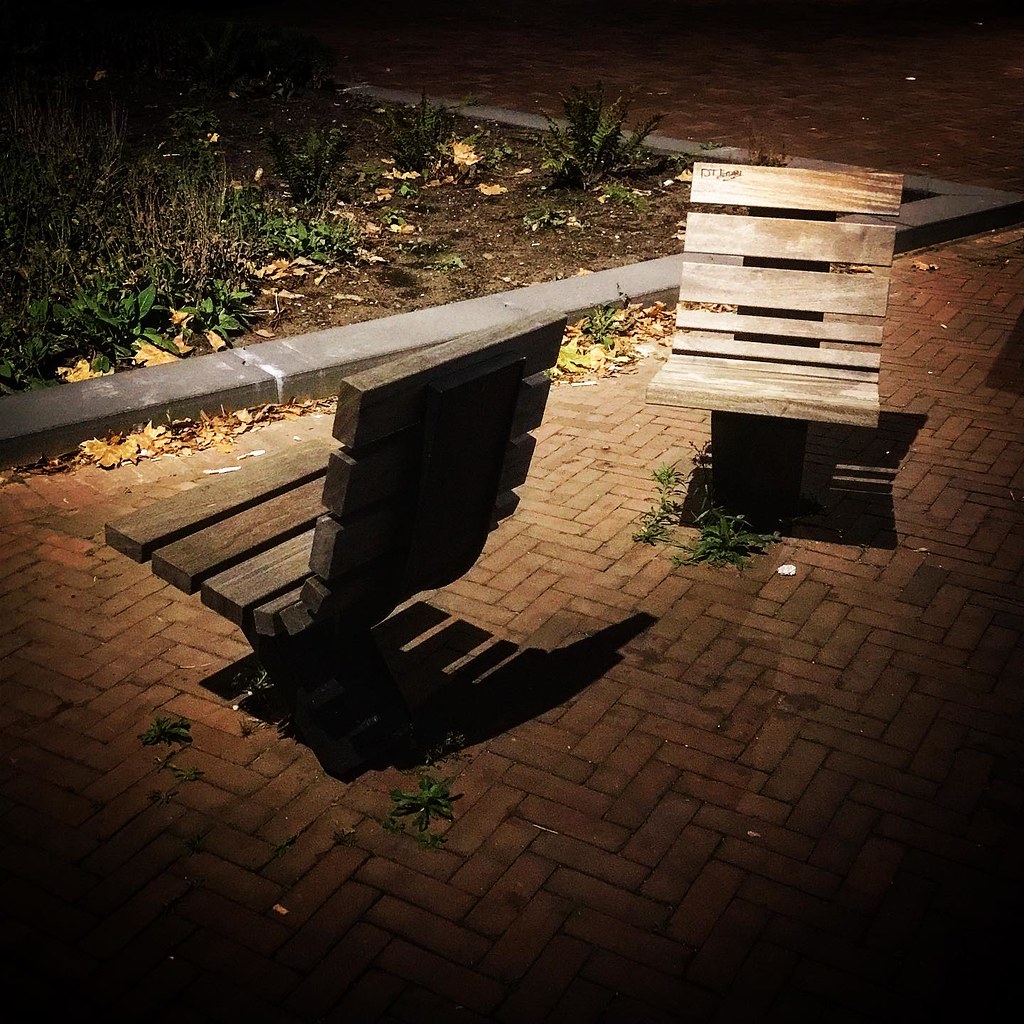The image depicts a nighttime scene illuminated by a street lamp, which casts a bright light on two single-seat park benches situated in the middle of the frame. These wooden bucket-style seats, appearing slightly distressed with medium brown planks, rest atop a concrete ledge that borders a poorly maintained garden area. The garden, primarily composed of dirt with a mix of dead plants and sparse green foliage, is encircled by a gray concrete border. The surrounding pathway or patio, likely made of interlocked bricks, shows signs of neglect with visible weeds sprouting through the gaps and a few pieces of garbage scattered on the ground. Shadows obscure the bases of the seats, making it unclear how they are mounted.